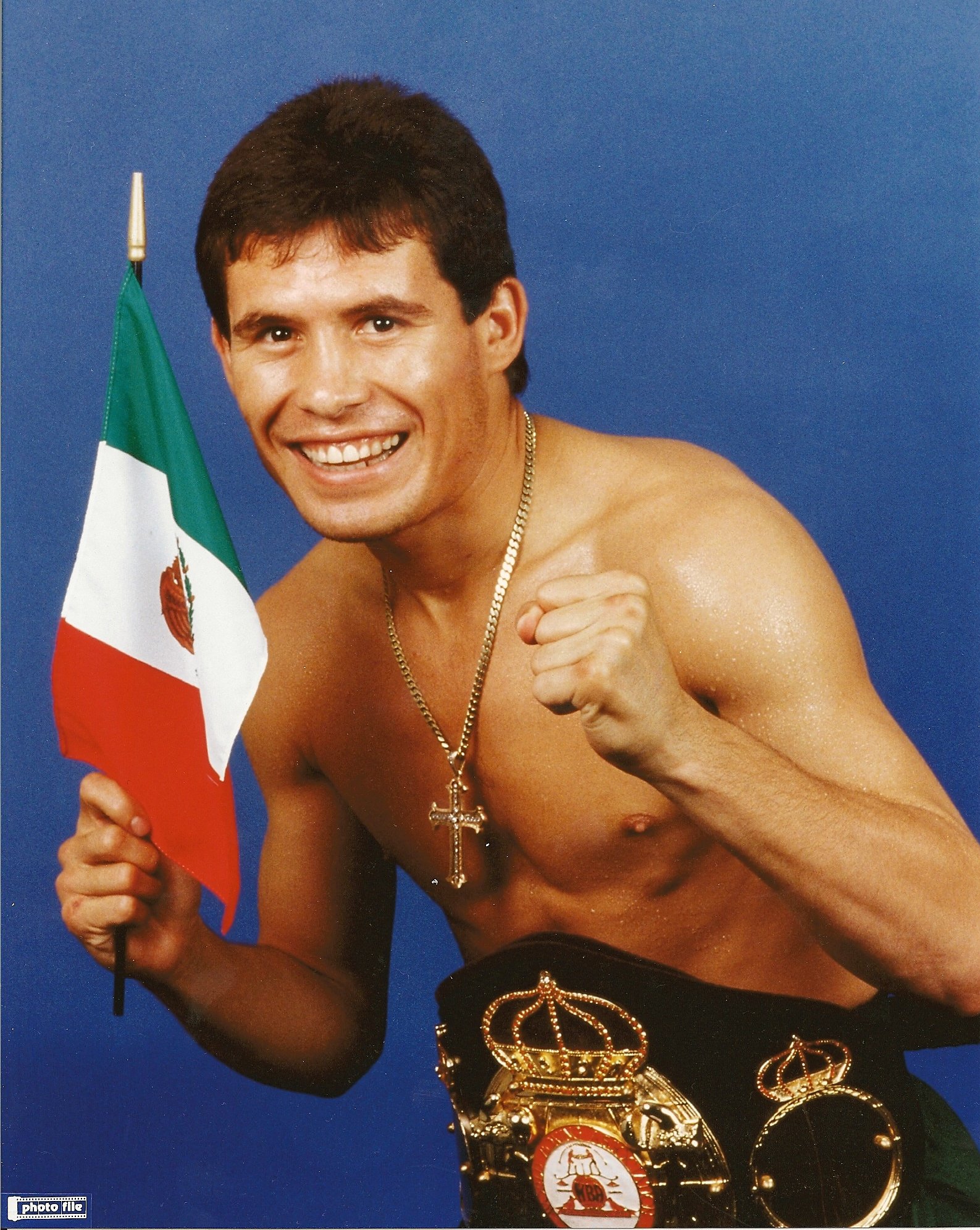In this vintage-style photograph of renowned boxer Julio Cesar Chavez, he is shown shirtless, smiling broadly with dimples accentuating his light brown eyes and thick eyebrows. Chavez’s short brown hair complements his approachable expression as he raises both fists in a fighter’s stance. In his right hand, he holds the Mexican flag, displaying its green, white, and red colors prominently despite an unreadable icon on it. Around his neck, a gold chain adorned with a jeweled crucifix dangles gracefully against his bare chest. He wears a distinctive black championship belt that features a golden crown atop a globe at its center, which signifies his athletic prowess and achievements. To the right of this main emblem, a smaller crown surrounded by a ring is visible, contributing to the belt's ornate design. The blue background contrasts well with Chavez’s figure, making his outlined features and details stand out. An inset image in the lower left corner, overlaid with white text, reads "photo file," adding to the photograph's nostalgic, film-like quality.